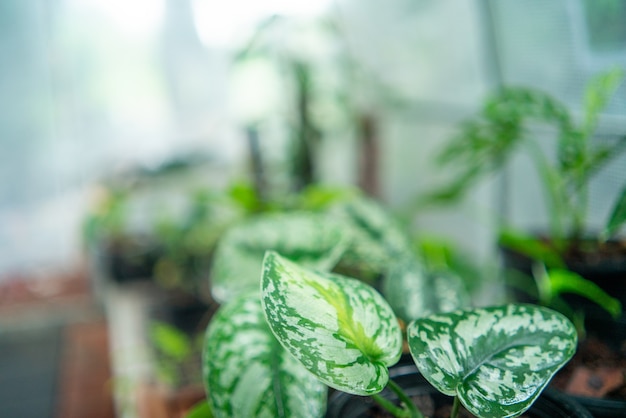The image features a close-up of three predominantly green leaves with intricate white splotches and specks, positioned in the lower center and lower right of the frame. The veins of these leaves are visible, with the central vein on one leaf being distinctly green, while the other shows a yellow vein. The leaves are wide and detailed, showcasing a clear, vivid texture. In the background, a blurred array of the same kind of plants extends, hinting at a horizontal layout with a window, some plant pots, and various plant accessories subtly visible but out of focus. The surrounding colors in the blurred background range from greens and whites to some red hues, primarily on the left side. The overall composition draws attention to the sharp details of the leaves in the foreground, making them the focal point against a softly blended backdrop.